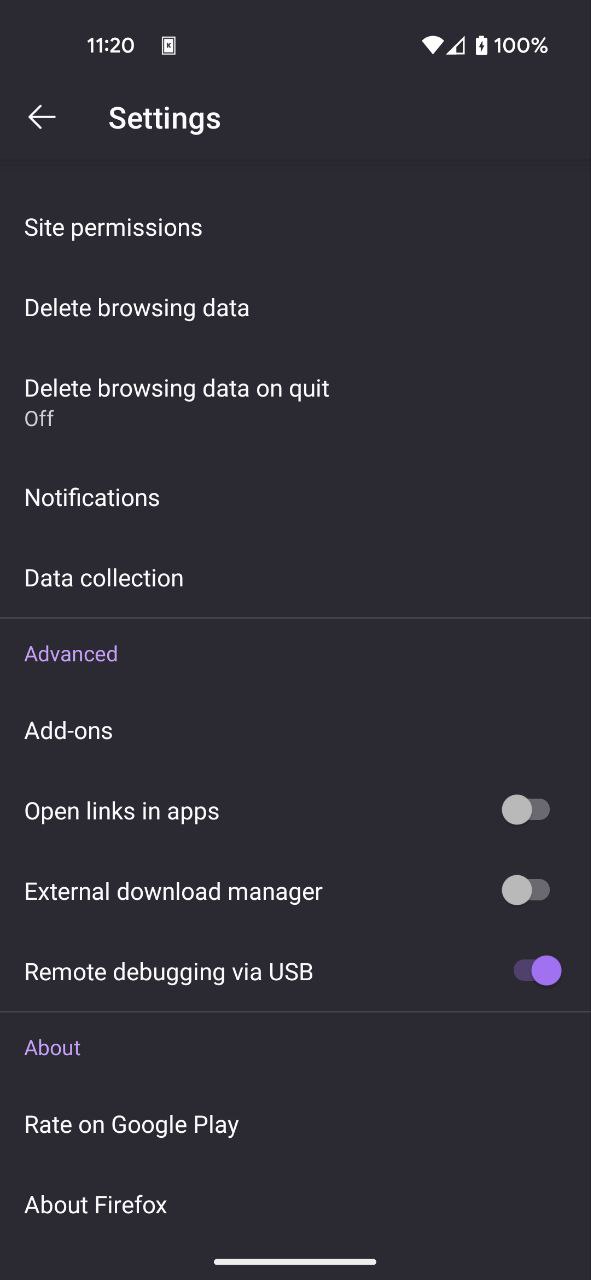The image is a detailed screenshot of a smartphone settings page, displayed in portrait mode with a dark blue to black background. At the very top of the screen, the time is shown as 11:20 AM, accompanied by a notification icon with the letter "K" inside a white square. On the upper right corner, indicators for Wi-Fi, service signal, battery status, and battery percentage (100%) are clearly visible.

Positioned below the time on the left-hand side, the screen displays "Settings" in white text next to a back arrow. Following this, a list of options is presented in white text, including "Site Permissions," "Delete Browsing Data," "Delete Browsing Data on Quit" (set to "Off"), "Notifications," and "Data Collection." A horizontal line separates these from additional settings.

Further down, in purple text, is the word "Advanced," which is followed by more options in white text such as "Add-ons," "Open Links in Apps" with a toggle switch set to off, "External Download Manager" with its toggle switch also off, and "Remote Debugging via USB" with its toggle switch turned on. Another horizontal line separates these from the final section.

At the bottom of the screen, in purple text, it says "About," followed by options in white text: "Rate on Google Play" and "About Firefox." Additionally, a short white horizontal line is centered towards the bottom of the screen, concluding the displayed settings options.